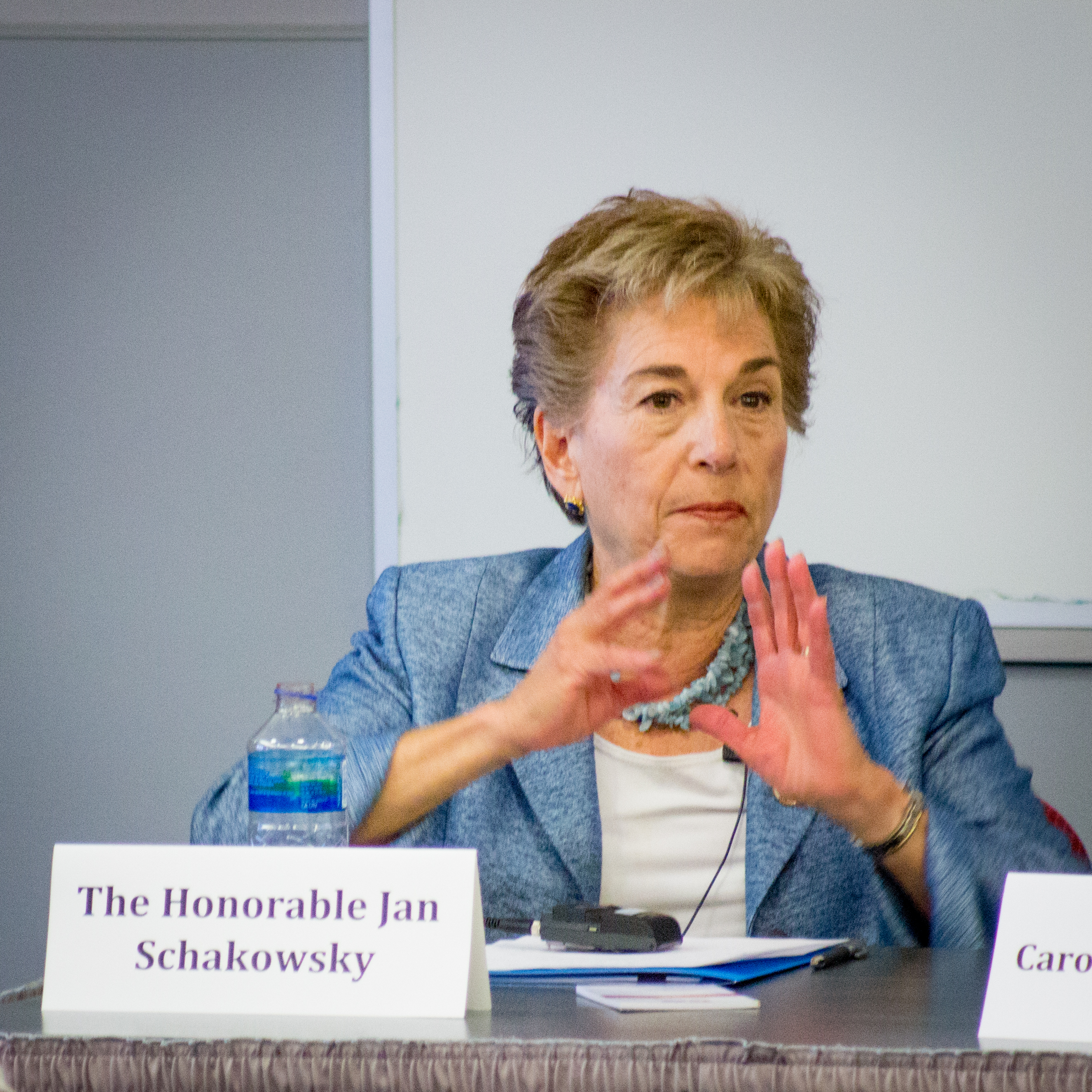This detailed photo features the Honorable Jan Schakowsky seated at a table adorned with a gray tablecloth and a gray curtain along its edges. In front of her, on the table, is a name card that reads "The Honorable Jan Schakowsky" in blue letters. To her right, another name card suggests the presence of additional speakers, although the other person is not visible in the frame.

Jan Schakowsky is captured mid-gesture, with both her hands raised as she speaks. She is dressed in a gray blazer jacket paired with a white undershirt and adorned with what appears to be a green frilly necklace. Her short, light brown-blonde hair and brown eyes are prominently visible, along with a notable blue studded earring trimmed in gold in her visible ear. 

On the table in front of her, there is a stack that includes a binder, some papers, a pen, and a walkie talkie positioned either on or near the papers. To her left is an open water bottle. She is seated against a backdrop that includes a whiteboard with no writing on it, situated against a gray wall.